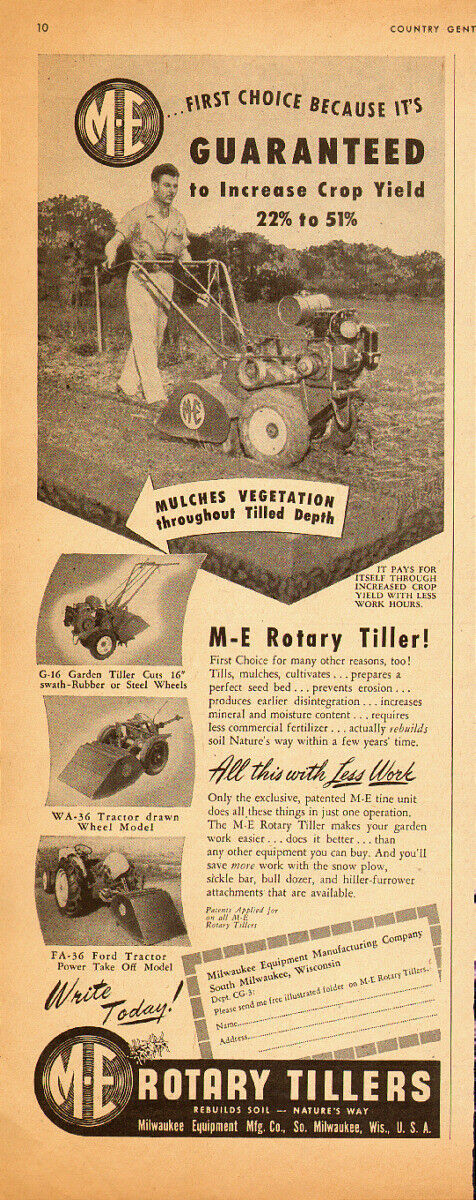The image is an old newspaper advertisement featuring the M.E. Rotary Tiller. The aged paper has turned brownish and discolored, giving it a vintage look. At the very top of the ad, there's the number "10," and on the top right, "Country Gent" is displayed. Prominently, a black circle with the letters "M.E." inside is visible, accompanied by the text, "First choice because it's guaranteed to increase crop yield 22% to 51%." 

Below this, a black-and-white photograph portrays a man operating a tiller with a large motor and substantial wheels, mulching vegetation throughout the tilled depth. Along the left-hand side of the ad, there are three additional images depicting different configurations of the equipment. Text beside these images reads, "M.E. Rotary Tiller," and in cursive script, "All this with less work."

The right-hand side contains two paragraphs of detailed information about the tiller. Towards the bottom, a small rectangular box suggests readers can "write today" for more information or to request the tiller. The lower section of the ad showcases a circle with "M.E." inside, next to the text "Rotary Tillers," and concludes with "Milwaukee Equipment Manufacturing Company, Milwaukee, Wisconsin, USA."